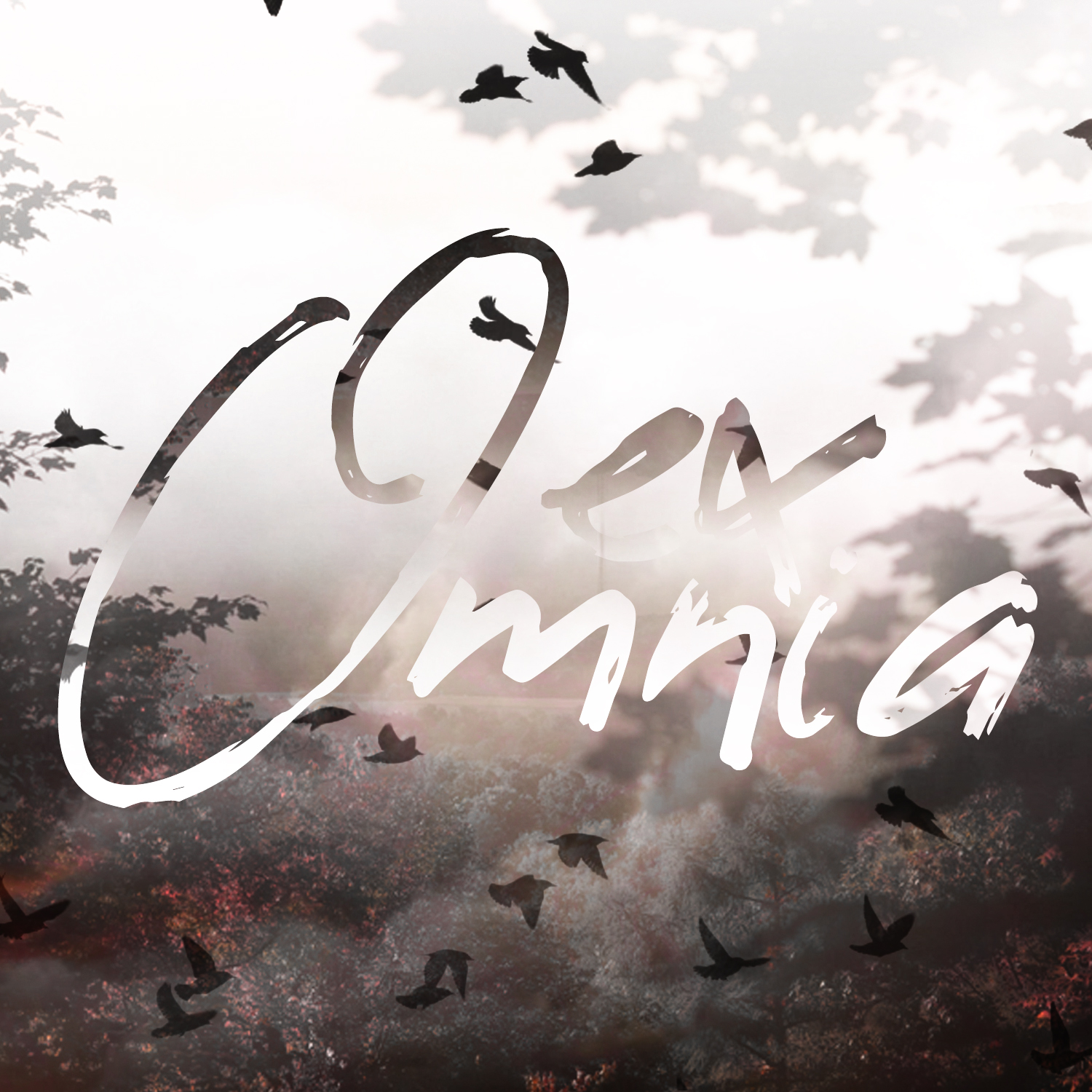The image is an artful blend of multiple photographic layers creating a surrealistic landscape. In the distant background, a pole is faintly visible, overlaid by silhouetted tree branches and leaves in dark gray tones. Scattered across the scene, a flock of black silhouettes of birds—likely crows or ravens—are in mid-flight, giving a sense of motion and life. A distinctive layer of semi-transparent green plant life overlays another layer featuring various trees and shrubs occupying the bottom foreground, evoking a sense of depth. The composite scene is tinted with diverse colors, including black, gray, white, red, orange, blue, and green, enhancing its dynamic feel.

Centrally positioned in the image is elegant cursive text reading "EX," immediately below which are the capital letters "O," "M," "N," "I," "A," forming "X Omnia." This text partially blends with the background through a transparency effect, enriching the visual complexity. The entire composition, with its integration of nature elements and text, suggests an outdoor wilderness setting, rendered with photographic realism and enhanced by special effects filters. The scene's overall feel is that of a meticulously crafted digital poster or web-based graphic, designed to elicit contemplation and wonder.